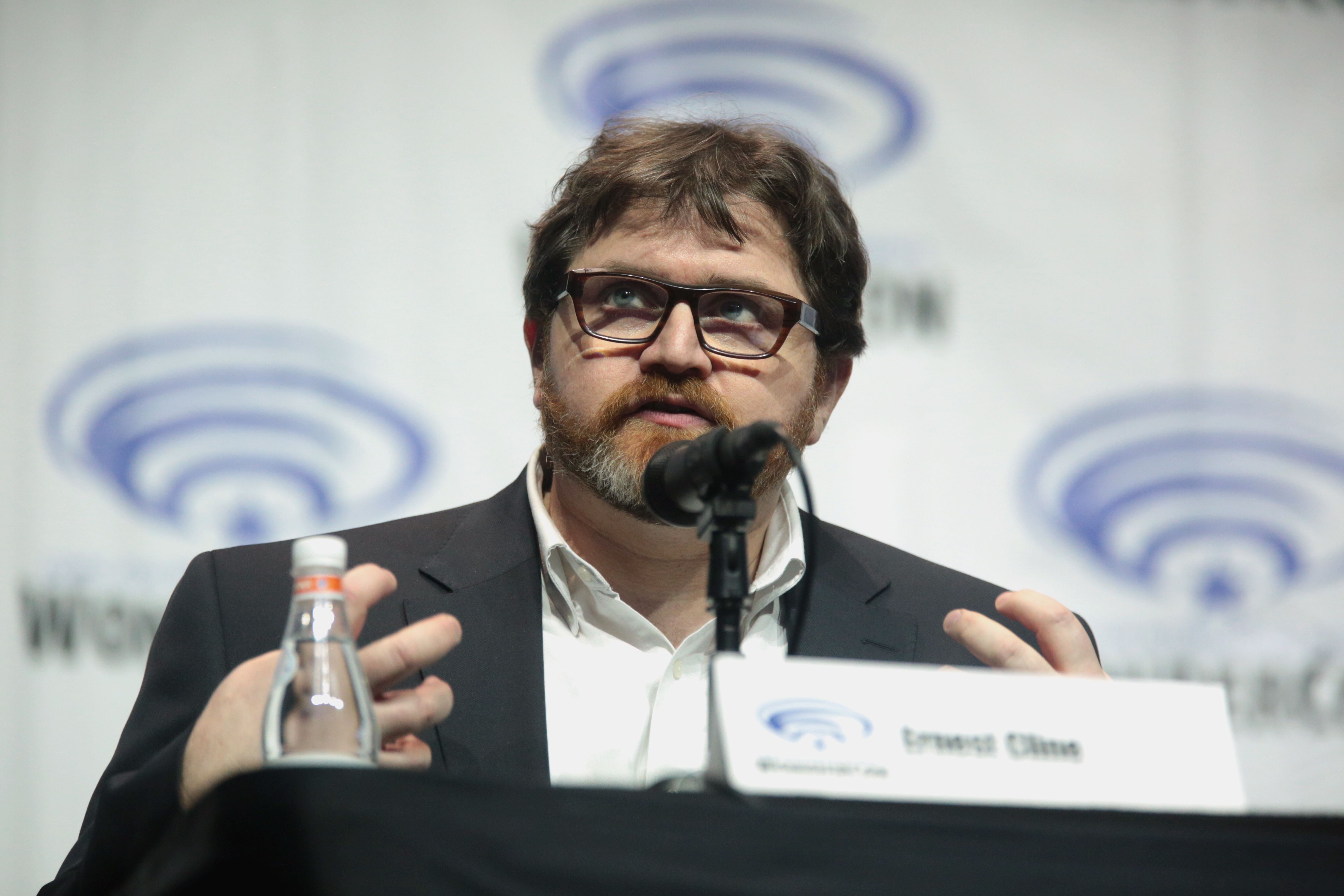In this image, a man in his 40s is passionately delivering a speech at a conference. He stands at a centrally located podium, which is draped with a curtain or cloth and equipped with a black microphone. Gesturing empathetically with both hands in a claw-like formation towards his chest, he emphasizes his points. Directly in front of his right hand lies a bottle of water, and a name tag is slightly out of focus below him on the podium. The man has tousled short brown hair and wears thick, dark brown plastic-rimmed glasses that frame his blue eyes. His beard is a mix of brownish-red with flecks of gray, giving him a distinguished look. Dressed in an olive-gray suit coat over a white button-down shirt with the top button undone, he exudes a professional yet relaxed demeanor. The backdrop features blurry, indistinguishable posters and signage, enhancing the atmosphere of a formal conference setting. The overall scene is captured indoors, creating a focused and intent ambiance as the man looks up towards the upper left corner, likely engaging with something or someone off-camera.